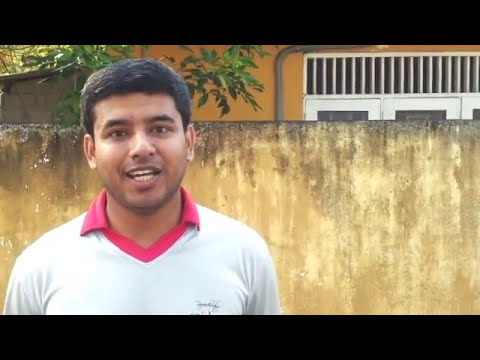The photograph captures a brown-skinned man with short black hair, who appears to be of Indian or Pakistani descent. He is positioned on the left side of the horizontal, letterboxed image, with the frame extending from the middle of his chest to the top of his head. The man, who is in mid-speech with his mouth open and teeth showing, is clad in a white shirt layered over a red collared shirt, with the collar neatly protruding over the top. Behind him, there is a large, brownish-gray stone wall, which partly obstructs the view of an orange building featuring white windows or doors. Additionally, green leaves from a tree are visible above the wall on the left-hand side, suggesting an outdoor setting.